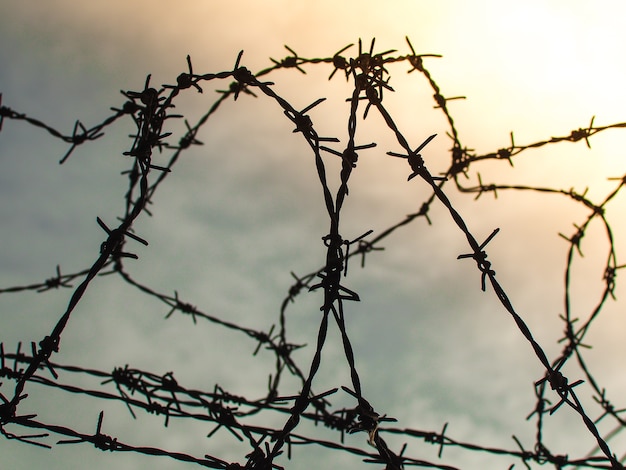This photograph, taken in landscape orientation, features an intricate close-up of barbed wire set against a cloudy sky backdrop. In the lower section of the image, three rows of taut, straight barbed wire stretch diagonally from the lower right to the lower left corner, slightly rising at the latter end. Above these straight rows, an elaborate entanglement of barbed wire loops and twists around itself, creating a complex pattern of pointy tines. The sky in the background is predominantly gray, with clouds that transition into a pinkish hue near a bright white area in the upper right corner, suggesting sunlight breaking through. The overall scene is a striking contrast between the dark silhouettes of the barbed wire and the softly textured, color-shifting sky.